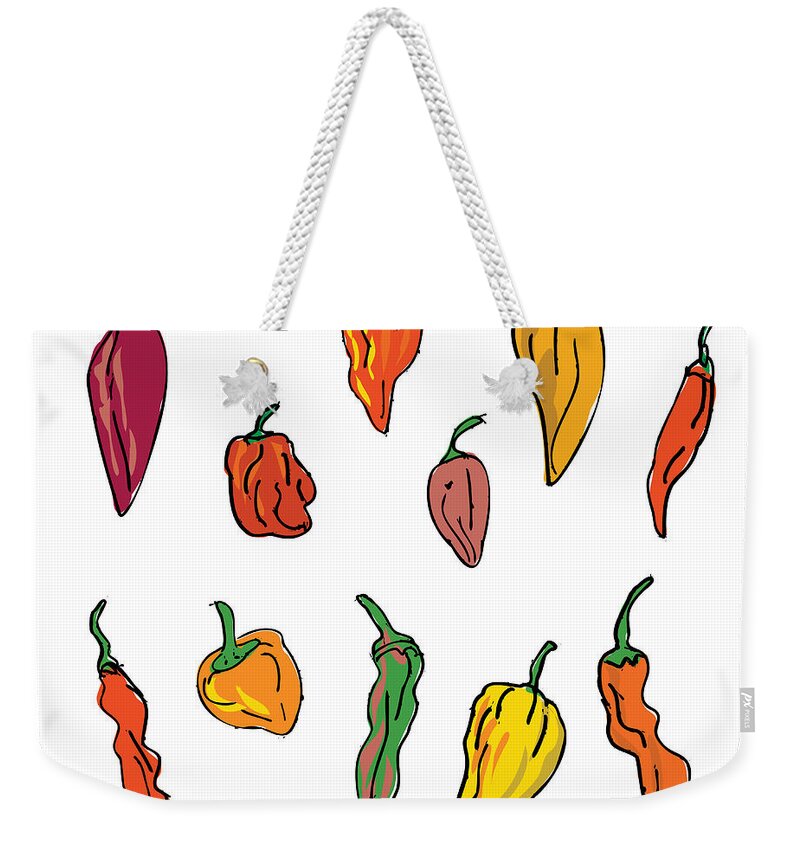This image features a small, white, canvas tote bag adorned with a distinctive pattern of various peppers. The bag has white, rope-like handles threaded through gold rivets at the top, forming an attractive and functional upside-down V-shape. The peppers, painted on the white canvas material, are arrayed in two distinct rows, showcasing an array of colors and shapes, including dark red, reddish-orange, brownish, yellow, green, and orange chilies. These peppers, which resemble different varieties such as Carolina Reapers and sweet Thai chilies, are depicted with black outlines and filled in loosely with vibrant colors. The corners of the rectangular-shaped bag are slightly rounded, adding to its unique aesthetic. Despite the somewhat sloppily drawn nature of the peppers, their distinct and colorful presentation makes the bag eye-catching. The design is displayed on a white background, emphasizing the bag's clean and artistic appearance.